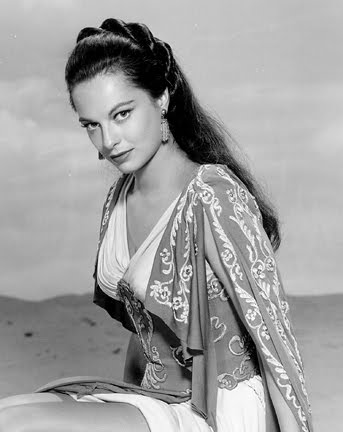This black-and-white photograph captures a woman set against what appears to be a backdrop of dirt or sand with possibly a cloudy sky. She is facing the camera, her head slightly tilted to the left, capturing three-quarters of her face. She has long, dark, tousled hair that is intricately braided or designed at the top, flowing down her back. Her earrings are long and rectangular, adding a touch of elegance. She wears a low-cut, V-neck white blouse or dress, adorned with tassels or a small button at the center, complemented by a draped, chiffon-like overgarment with a subtle white pattern that falls over her shoulders, revealing parts of her arms. Her lower garment appears to be white shorts or a skirt. The photograph exudes a serene and contemplative mood, accentuated by her direct gaze at the camera and her subtly made-up face, suggesting a professional photoshoot ambiance.